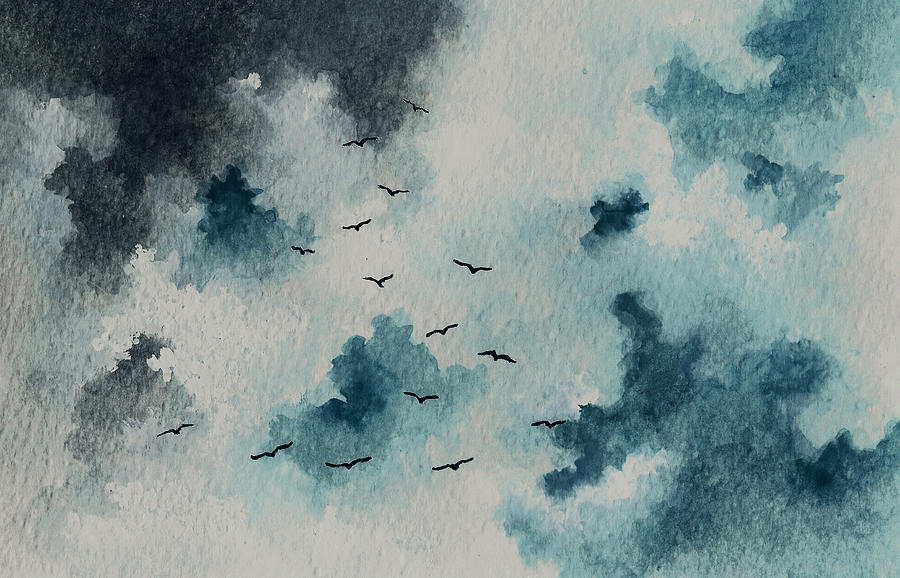This artwork appears to be a watercolor painting on a white or beige canvas, possibly seeping through in some areas. It primarily depicts a sky scene, with a soft and impressionistic style. The dominant colors are varied hues of blue and teal, along with whites, blacks, grays, and hints of beige. The sky is adorned with white clouds and darker, inky blue regions, particularly in the upper left corner, indicating storm clouds. Central to the painting is a flock of 10 to 15 birds, reminiscent of seagulls, depicted with simple black lines and flying close together towards the center of the image. Notably, there's a dark green, wavy mass in the upper left corner that could be a storm cloud or even a tree, blending indistinguishably with the bluish-green backdrop, suggesting either additional trees or variations in the sky. The overall scene creates a sense of dynamic motion and a blend of natural elements, masterfully captured in the flowing strokes of watercolor.